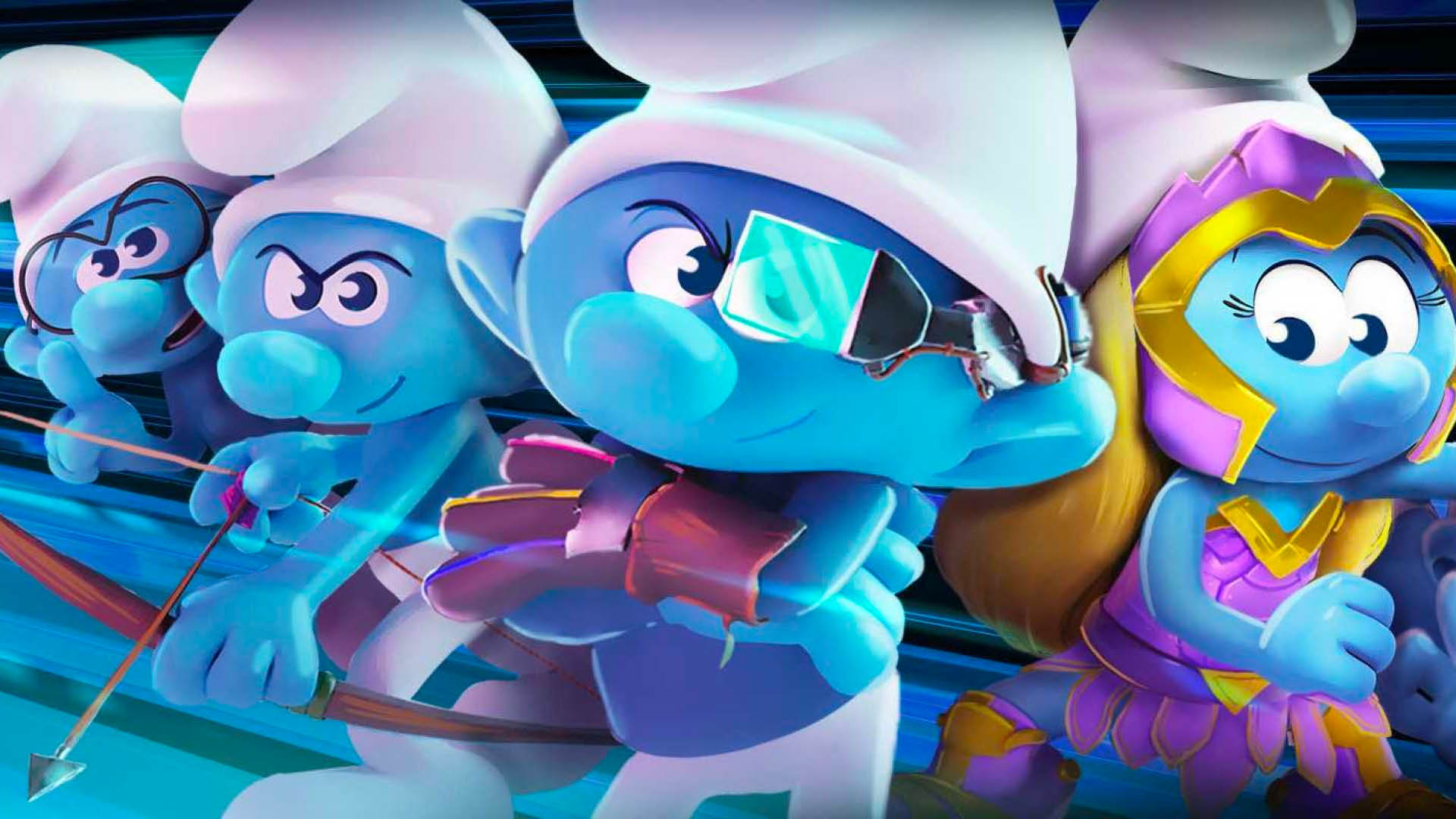This vibrant illustration features four iconic Smurf characters, all with blue skin, white pants, and drooping white caps. Standing in a row, the Smurfs appear poised for action, reminiscent of a scene from a new Smurfs movie.

Papa Smurf, positioned on the far left, is identifiable by his glasses and studious demeanor, raising a finger as if imparting some crucial wisdom. Next to him is a Smurf with furrowed eyebrows, holding a bow and arrow, projecting a sense of readiness for battle. The third Smurf, positioned closest to the viewer and the largest of the group, sports an augmented reality headpiece over his left eye, resembling Google Glass, complete with an intricate setup of colored wires—purple, yellow, and pink—attached to a maroon glove, signaling his high-tech role.

On the far right stands Smurfette, distinguished by her Amazonian-inspired gold and purple armor and long blonde hair. Her outfit includes a breastplate and a Greek-style headpiece, adding a touch of heroic elegance to her appearance. Together, these Smurfs, adorned in their unique gear, evoke a sense of an impending adventure or battle, integrating both traditional and modern elements into their ensemble.